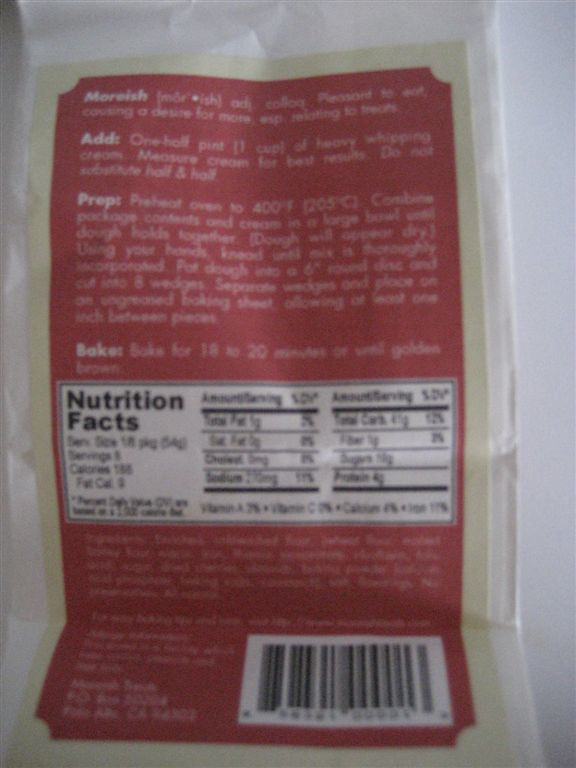This color photograph captures the back of a food package. The packaging is red with detailed white text encompassing various sections. At the top, instructions for meal preparation are written in white text, providing specific directions such as adding one half pint (one cup) of heavy whipping cream, measuring the cream for best results, and baking for 18 to 20 minutes until golden brown, cautioning not to substitute with half and half. The middle section prominently features a horizontal white rectangular box containing black text that details the nutrition facts, listing contents like energy, sugar, and protein levels. Additionally, information about the company is present on the package. On the bottom right, there's a distinct white background with a black barcode. Although the photo is somewhat blurry, it's evident that the text is printed on a red rectangular label, which suggests it might be a ready-made meal package that requires baking.